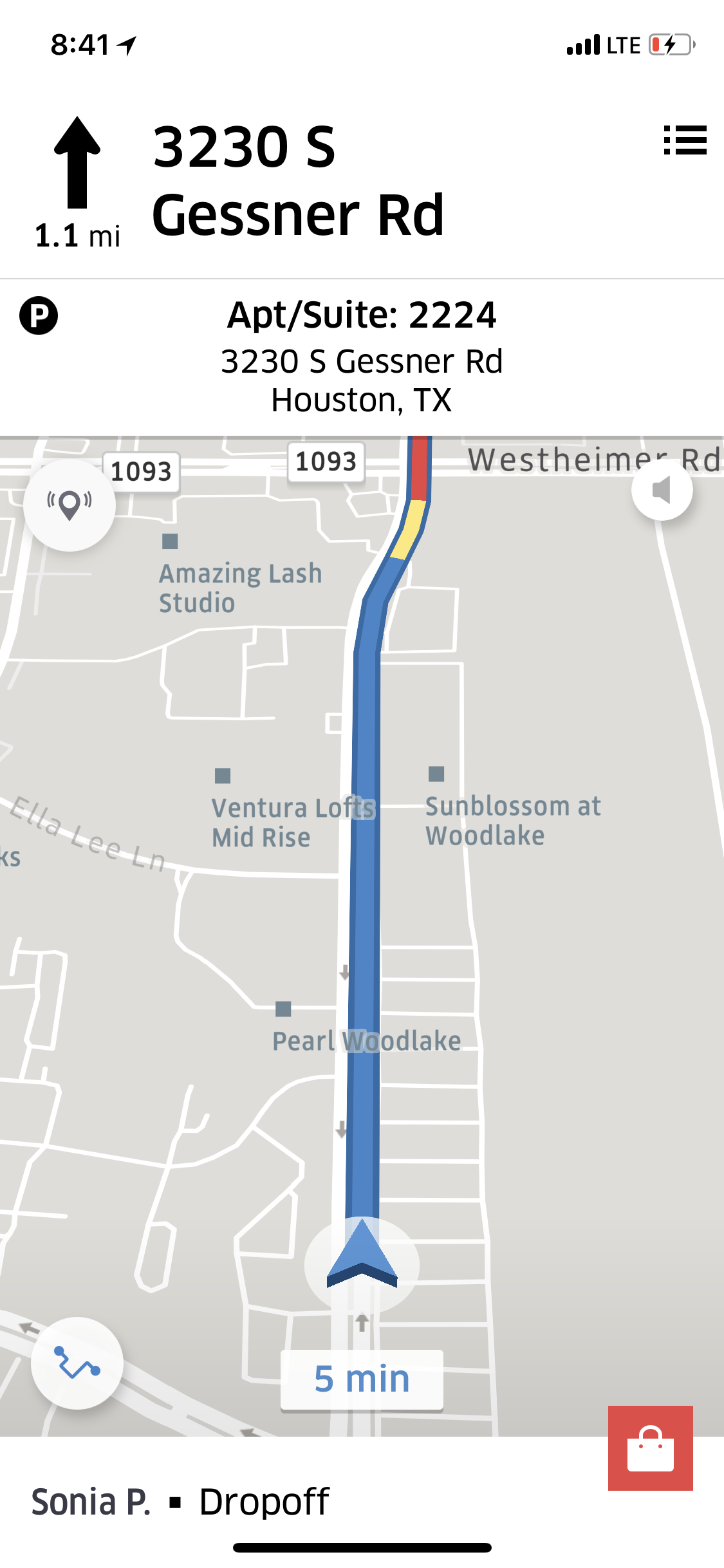This is a vertically rectangular screenshot from a cell phone, depicting a map interface with navigation details. At the very top of the screen, the phone displays the current time as "8:41," the cellular status as "LTE," and the battery icon shows a low battery marked in red. Below this, the map shows a blue route starting from the bottom, labeled "5 minutes" with a straight arrow pointing ahead, indicating a 1.1-mile journey. The route traverses through different areas, marked in blue, yellow (indicating slowdowns), and red (indicating heavy traffic). Prominent on the map is the address "3230 South Gessner Road," with additional detail specifying "Apartment Suite 2224, Houston, Texas." The bottom of the screen features the text "Sonia P. - Drop off," suggesting a rideshare context, and a small shopping bag icon is visible in the bottom right corner. The background of the map screen is gray.